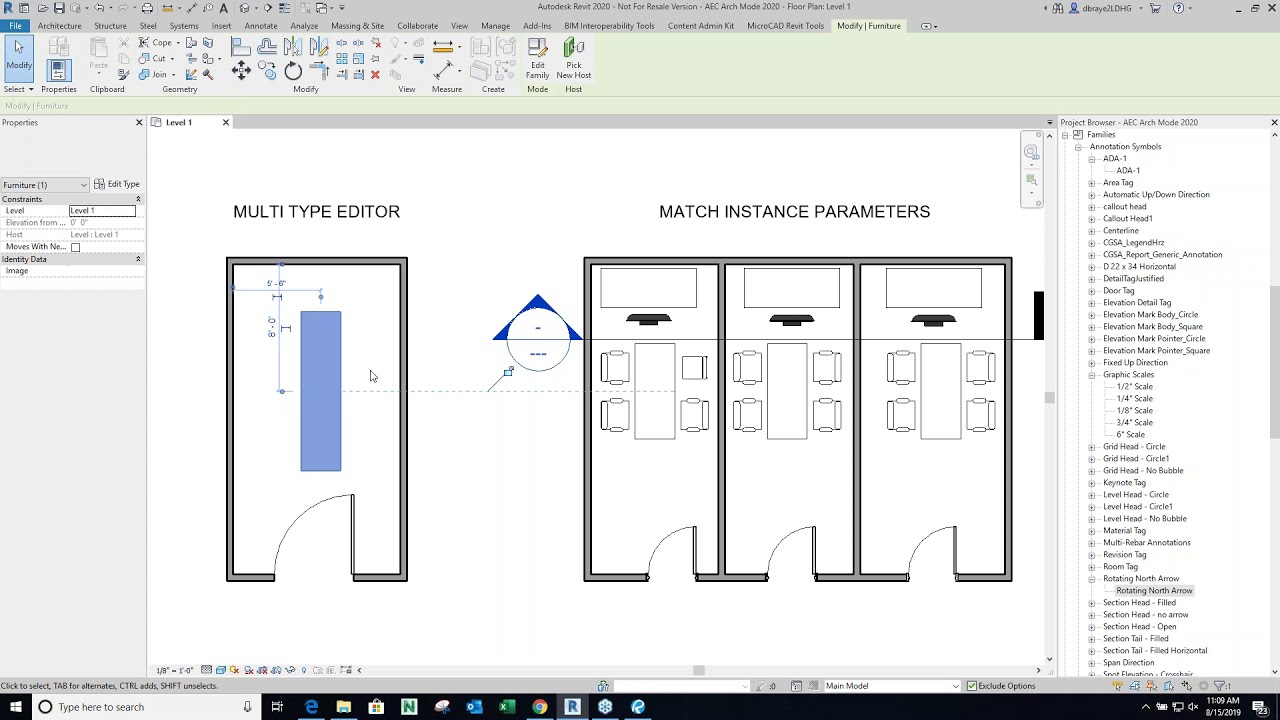The image is a screenshot of a computer application showcasing a detailed architectural design schematic. The interface appears to be a computer-aided design (CAD) application, although the specific software is not clearly identified. At the very top, there is a gray toolbar that includes standard window controls like minimize, maximize, and close buttons, along with various symbols and menu options arranged in a grid format.

The main section of the screen displays a white background divided into two columns. On the left, in black type, it says "multi-type editor" beside a section that includes an outlined gray rectangle representing a room with an open door at the bottom. Inside this room, there's a smaller blue rectangle with graph markings.

To the right, there is another labeled section that says "match instance parameters." This section contains three identical designs arranged side-by-side. Each design features a top-down view of an office room with a rectangular table and chairs, alongside what appears to be a TV or computer screen at the top. The rooms also have doorways at the bottom edge, swinging open from left to right, further adding detail to the schematic representation.